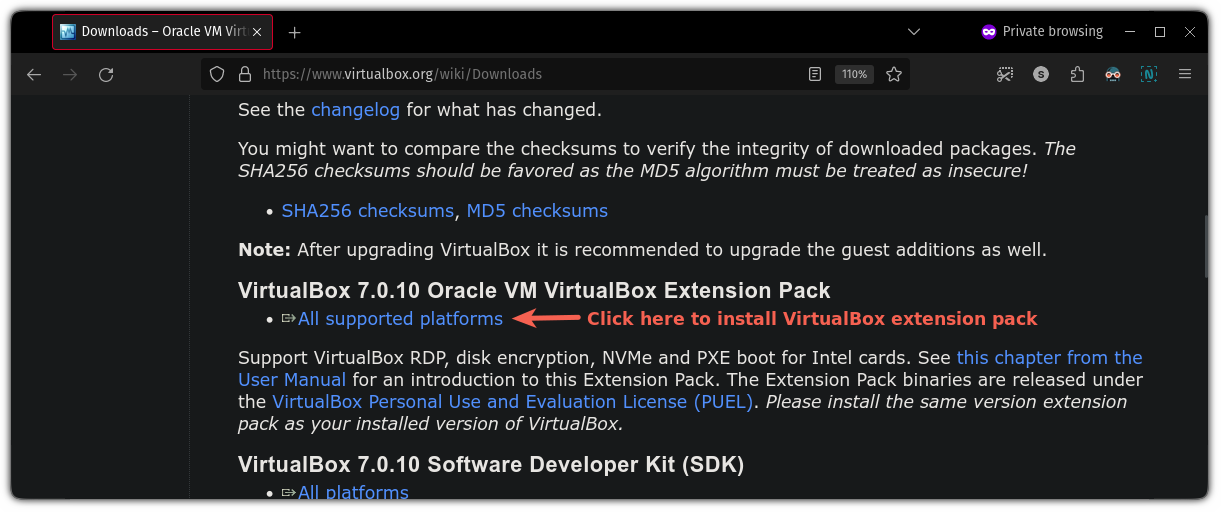In this screenshot of a web browser, the sole tab at the top left is labeled "Downloads Oracle VM Vert" and is highlighted with a blue square and a red outline. To the immediate right of this tab is a plus symbol icon for opening new tabs. The majority of the upper part of the screenshot is blank, but the top middle features a URL bar displaying "www.virtualbox.org/wiki/Downloads" along with a lock and shield icon to its left, indicating connection security. Further to the left are navigation icons, including a left arrow, a right arrow, and a refresh icon. On the top right of the screen, there is a "Private Browsing" label followed by window management icons: a dash for minimizing, a square for maximizing, and an X for closing the window.

The central part of the image contains text-heavy content. Key phrases in blue are highlighted, including "Changelog," "SHA-256 Checksums," "MD5 Checksums," "All Supported Platforms," "This chapter from the User Manual," "VirtualBox Personal Use and Evaluation License," "P-U-E-L," and "All Platforms." These links are interspersed among various paragraphs of text. A prominent red arrow pointing to the left is also present in the middle of the screen, directing attention to some significant element within the image.